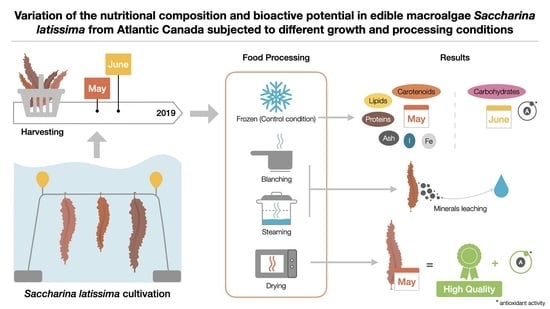The image depicts a detailed, computer-generated flowchart set against a solid white background, with a prominent black title at the top reading "Variation of the Nutritional Composition and Bioactive Potential in Edible Macroalgae Saccharina latissima from Atlantic Canada Subjected to Different Growth and Processing Conditions." The flowchart uses various colors to distinguish different sections and pathways clearly.

Starting at the bottom left, the flowchart begins with "Saccharina latissima Cultivation," illustrated by an image of plant leaves, and a subsequent section showing the leaves in a basket labeled with "May" and "June." Arrows guide the viewer from "Harvesting" through to "Food Processing" in the center, which is denoted by a rounded rectangle. The "Food Processing" section is divided into four methods: Frozen, Control Conditions, Blanching, Steaming, and Drying, each paired with corresponding images.

From the "Food Processing" rectangle, arrows direct to the right side of the flowchart, leading to a section named "Results." This results section is subdivided into three parts representing the outcomes of Frozen, Blanching plus Steaming, and Drying processes. The multicolored elements and clear flow structure highlight the sequence from cultivation through processing to the final results, providing a comprehensive overview of the nutritional and bioactive variations in the edible macroalgae.